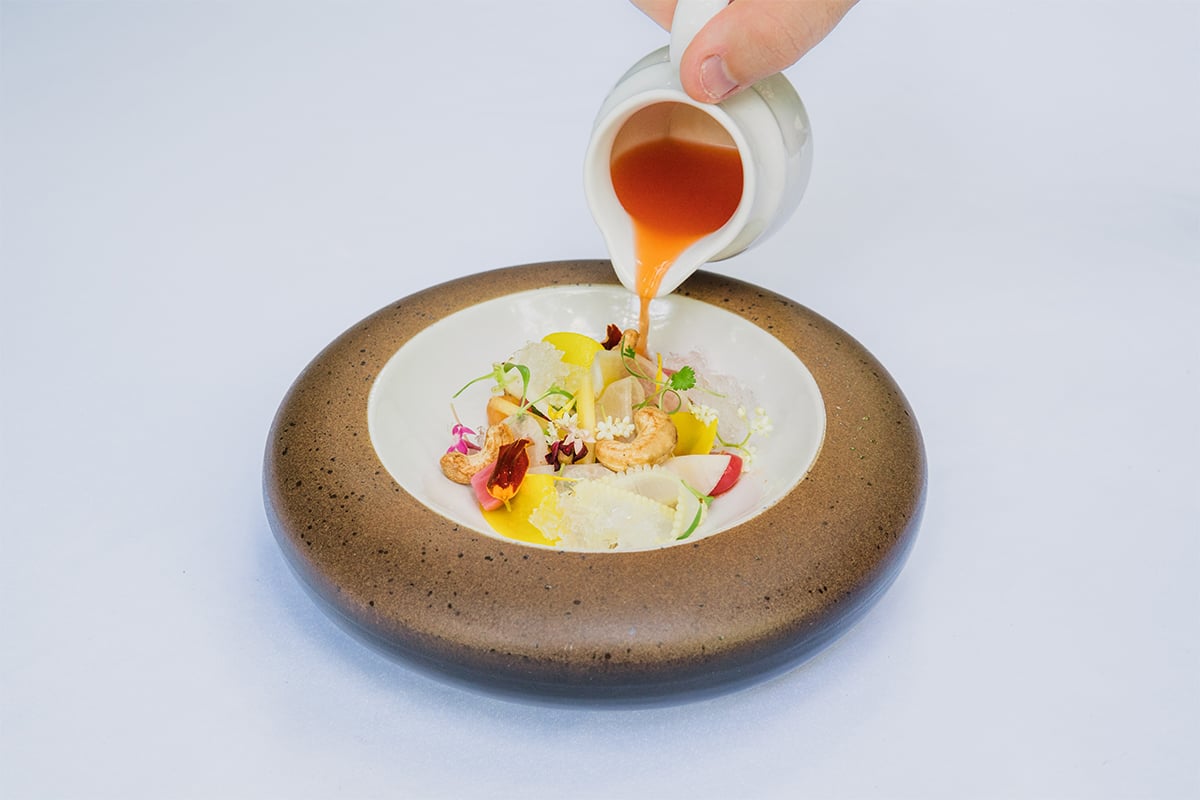This image captures a detailed scene of a meal presented in an elegant ceramic dish. The dish itself is sizable and robust, featuring a thick, brown rim with an indentation that houses a white, plate-sized center. Within this center plate rests a fine assortment of foods, suggesting a sophisticated gourmet creation, likely from a non-American cuisine. Visible items include slices of apple, pieces of banana, shreds of citrus which may be lemon, a couple of cashew nuts, and some delicate greenery that resembles parsley or other garnishing herbs. While some elements appear radish-like and others floral, the overall composition retains a sense of culinary artistry with a fruit-heavy focus. Adding to the visual appeal is a hand delicately pouring a thin, amber-orange or brown caramel-colored sauce from a small white ceramic pitcher. The pitcher itself has a subtle blue gradient fading into white. The background of the photograph is lavender, providing a serene and complementary backdrop to the vibrant dish.